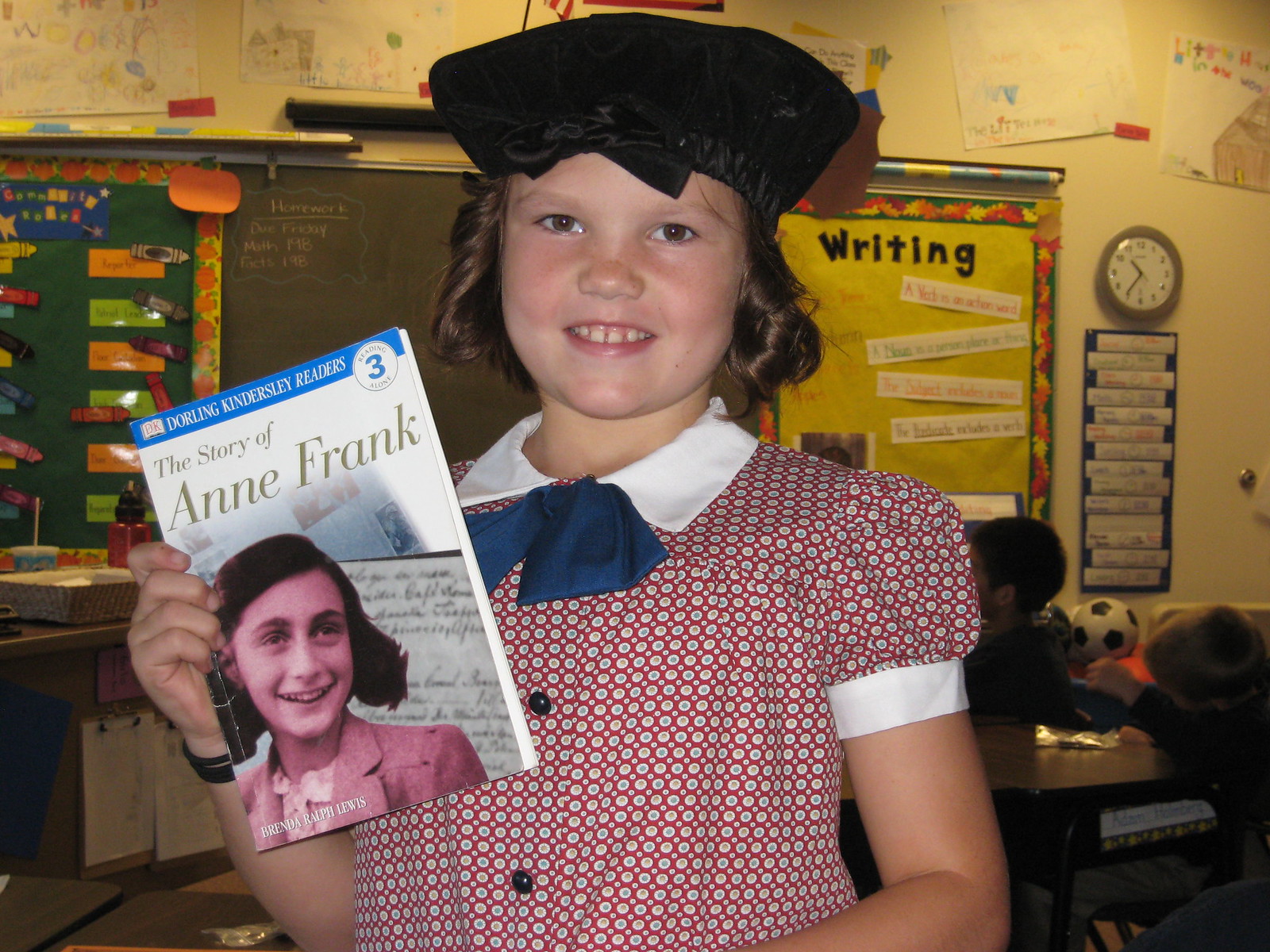In this large square photograph, a young girl, approximately 7 to 10 years old, stands at the center of a classroom looking directly at the camera and smiling. She has short, curly brown hair that frames her face and is adorned with a black hat featuring a bow at the front. Her outfit consists of a distinctive red and white patterned blouse with a white collar, blue bow tie at the top, and puffy short sleeves with white hems. She holds a book titled "The Story of Anne Frank" prominently in her right hand, which features a photo of Anne Frank on the cover, suggesting she might be dressing up as Anne Frank. The backdrop is a typical classroom setting with various elements visible: a chalkboard directly behind her, a bulletin board with writing next to it, and several white papers and posters hung on a beige section of the wall. There are also other students sitting at desks in the background, visible in the lower right corner. The classroom is filled with a mix of colors including red, white, blue, brown, yellow, green, gray, orange, tan, and silver. The overall ambiance suggests an indoor school setting in the middle of the day.